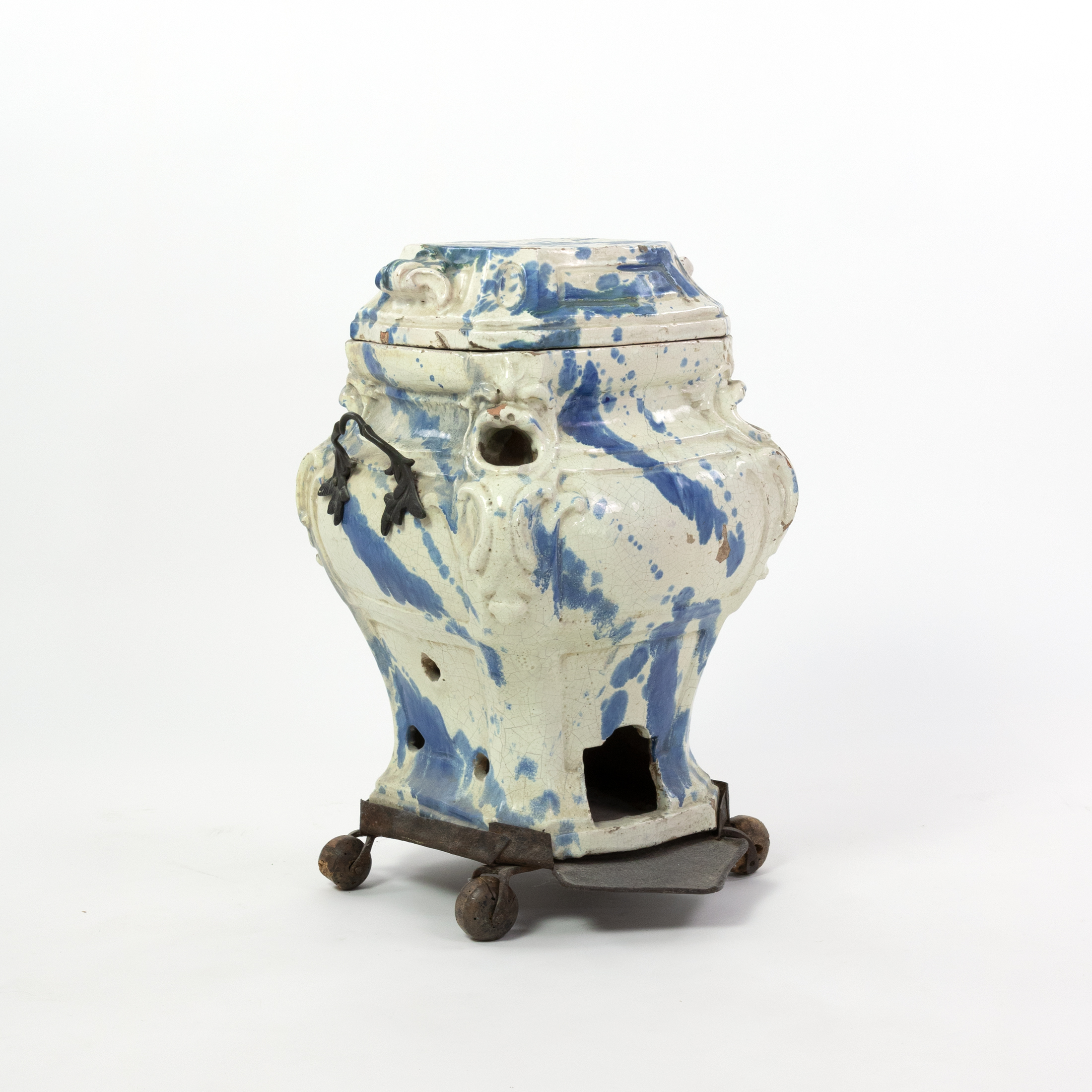The image depicts an intricate and antique-like porcelain vase, characterized by its off-white or shiny white surface adorned with diagonal blue streaks and occasional blue polka dots. The vase features a lid and several openings, or holes, on various parts of its structure, suggesting its historical use as an 18th or 19th-century stove, possibly referred to as a faience. This would have been used for heating rooms, with specific cut-outs potentially meant for kindling or other burnable materials. The vase is mounted on a robust black metal platform, which includes black metal handles and rolling casters for mobility. The overall setup is quite artistic, suggesting this item now serves more as a decorative antique. The professional photograph, slightly taller than it is wide, minimizes shadows and showcases the vase's glossy finish and historical craftsmanship.